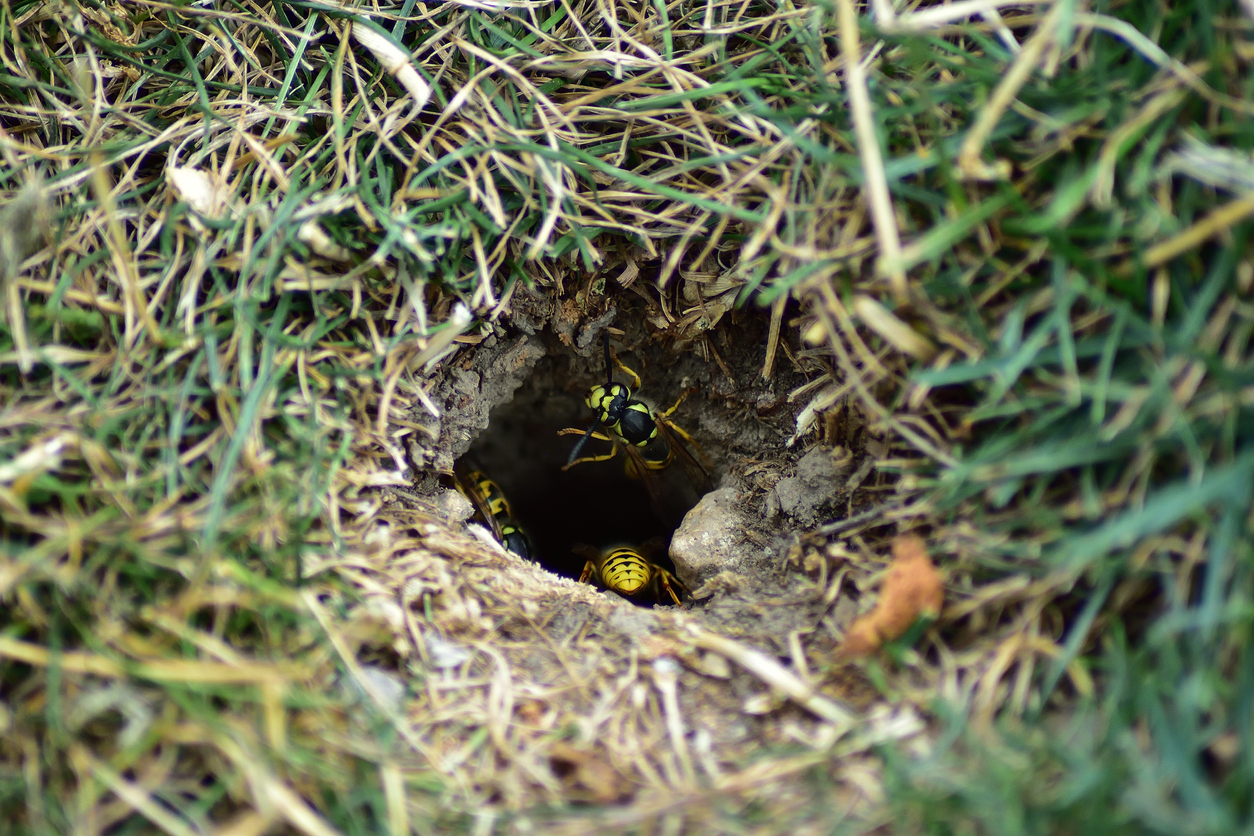This image is a close-up of a dirt hole in the ground, surrounded by a mix of green and dried beige grass. The scene captures a small, tightly framed section of the terrain, highlighting the underground burrow with meticulous detail. Three yellow and black dirt wasps, commonly referred to as yellow jackets, are visible within the hole. The wasps exhibit distinct black marks along their backs and faces, indicative of their species. One yellow jacket is positioned at the upper part of the hole, oriented upside down, with its head and back clearly seen. Another is at the bottom, showing mostly its thorax, while the third is slightly to the left, revealing its upper back. The dirt around the entrance appears mostly dry, though there are hints of moisture closer to the hole. Additionally, a small dried leaf can be seen towards the lower right side of the frame. The burrow is meticulously dug out, making it prominently visible amid the grass that appears to grow concentrically towards the opening. The setting conveys an active wasp nest but maintains a tranquil, natural ambiance as long as undisturbed.